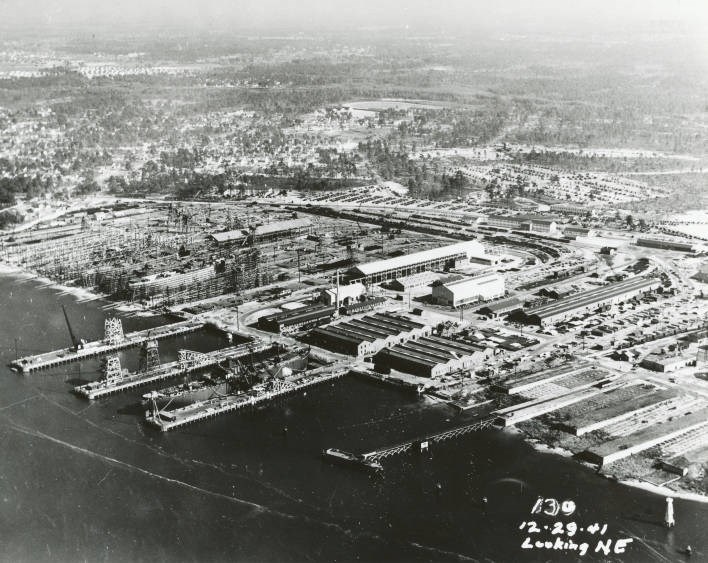A detailed aerial black and white photograph dated December 29th, 1941, shows a wintry scene of a port city, likely in New England, given the visible snow and the presence of water. The image is labeled "139-12-29-41 looking NE" at the bottom right corner. The landscape appears flat with no prominent tall structures; instead, it features many flat buildings and roads. On the lower left, a shiny black area suggests water with four long docks extending into it, possibly used for shipping cargo. A large ship is docked nearby. The upper portion of the photo reveals a cluster of buildings, bare ground, and scattered trees that appear as black dots due to the distance and haziness of the old photograph.